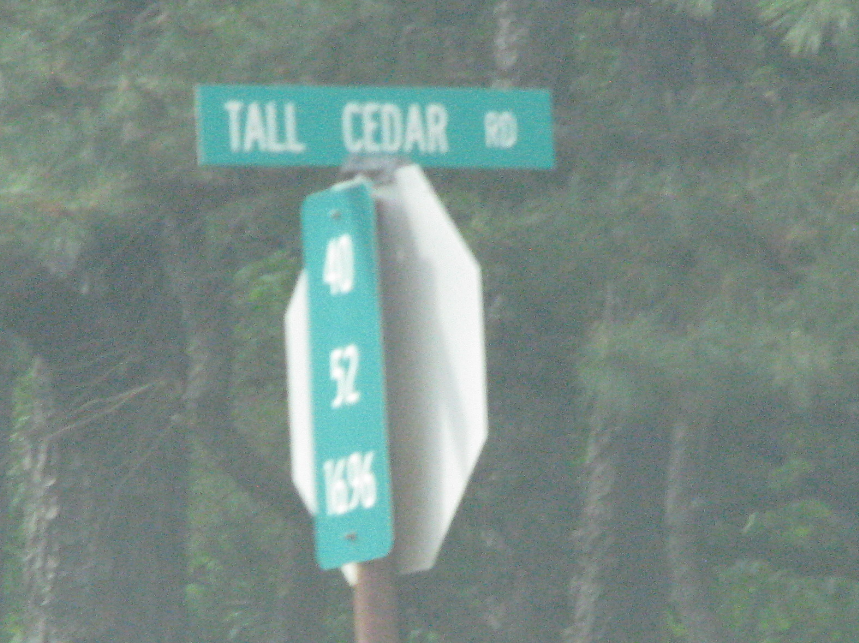In this hazy photograph, we observe a tall street sign positioned against a backdrop of lush, green trees with needle-like pine leaves and big brown trunks. The primary sign features a green rectangle with white lettering that reads "Tall Cedar Road." Mounted above and sharing the same pole is another green sign displaying the numbers 40, 52, and 1696 in white, arranged from the top to the bottom. The pole also supports an octagonal sign viewed from the back, revealing its white surface, indicative of a stop sign.